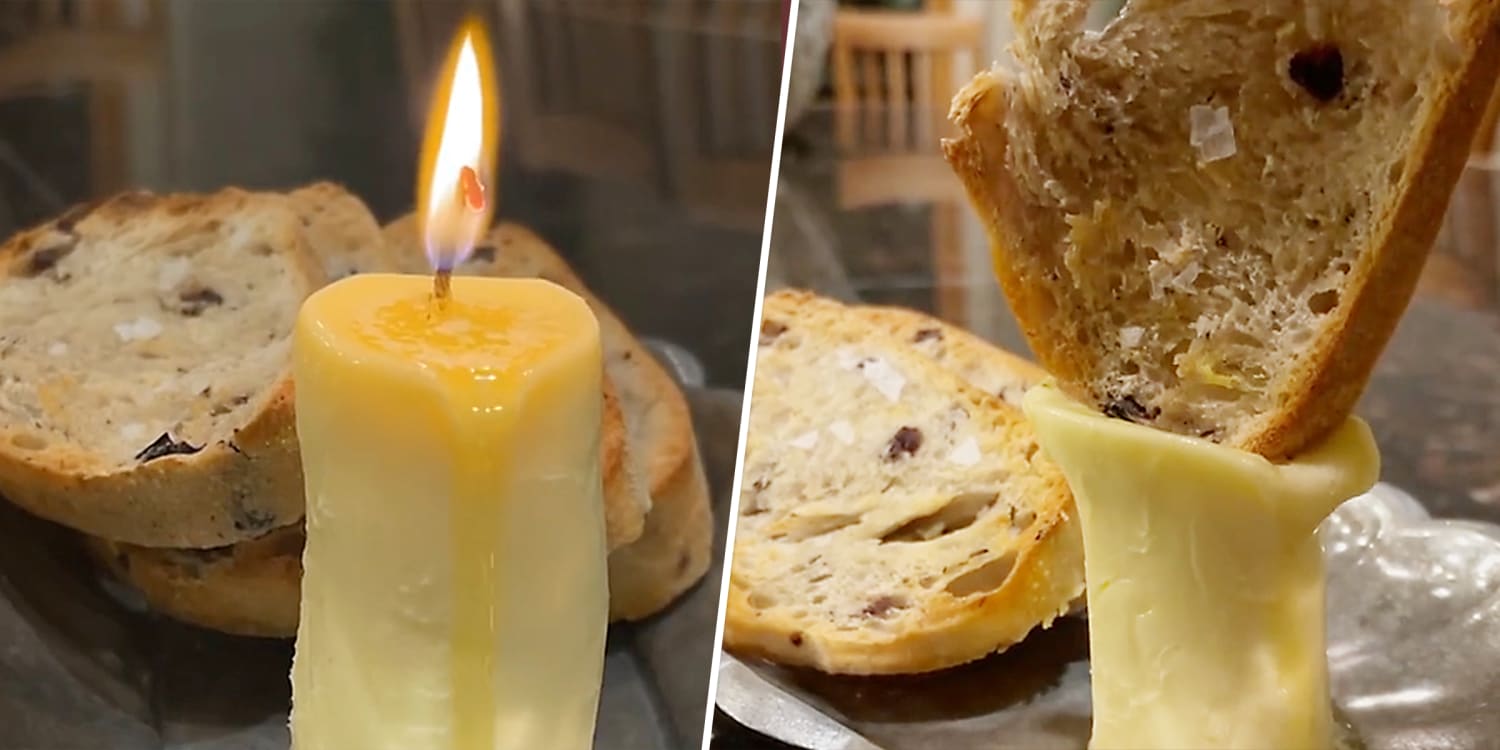This photographic indoor image is a diptych, divided by a diagonal white line, featuring two side-by-side photos with no text. The left photo displays a lit, yellow wax candle, somewhat misshapen with curvy sides and a glowing yellow flame, situated in front of two toasted slices of sourdough bread. The candle appears cylindrical but has deformed slightly due to the heat. Behind this setup is the blurry, out-of-focus back of a brown wooden chair, hinting at a restaurant-like setting.

In the right photo, the candle’s flame has been extinguished, as a piece of toasted sourdough bread has been pressed down into the softened wax, causing it to spread and adapt to the bread's surface. Another slice of sourdough bread rests on its side on the table. The background items from the first image are now more visible, confirming the setting includes wooden chairs, contributing to the homely, indoor atmosphere.